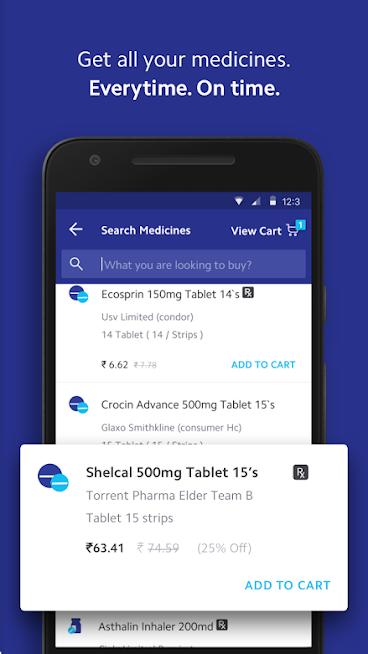A detailed graphic showcases a pharmacy app interface, set against a soothing blue background. The prominent feature is a realistic phone mockup, likely an Android device, displaying the app's medication search page. At the very top, a reassuring message reads, "Get all your medicines every time on time." The search bar on the phone screen awaits input, with placeholder suggestions including "Ecosprin 150mg tablet (14s)," "Crocin Advanced 500mg," and "Shell Cal 500mg." Prices are visible but in an unfamiliar currency. An inhaler, partially obstructed, appears near the bottom of the list. The top-right corner of the screen shows a shopping cart icon, indicating one item already added. In the immediate foreground of the image, another pack of "Shell Cal" seems ready to be added to the cart, capturing the essence of efficient and timely medication management.